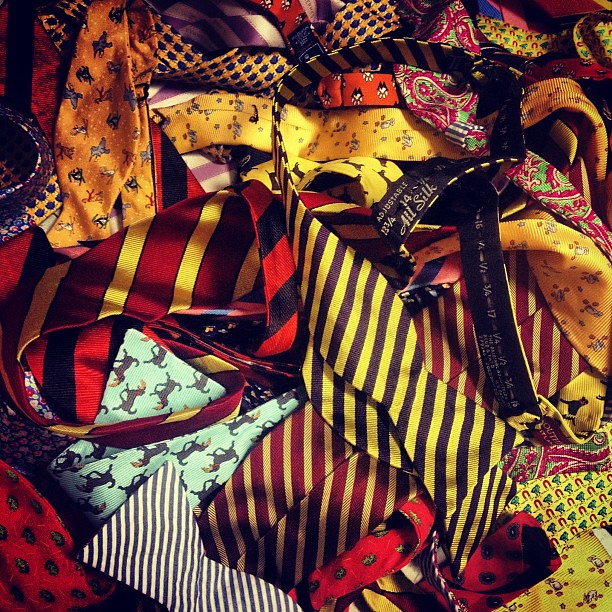This vibrant photograph showcases a chaotic assortment of colorful ties, each boasting unique patterns and textures. Dominating the scene are ties in a range of bright hues, such as striking yellows, vibrant reds, teals, purples, and cranberry. Close inspection reveals the intricate designs: near the center, a tie with bold yellow and black stripes catches the eye, adjacent to another striped tie with a striking red, black, and yellow combination. In the bottom left corner, a red tie is adorned with light green or gray paw prints, while directly above, a light green tie features black dogs clutching orange frisbees. Some ties display intricate paisley patterns with lime green and hot pink, and others feature animals against a blue background. Among the ties, one stands out with inscriptions such as "all silk," "adjustable, 13 and 3 quarter," and other measurements. The ties overlap and intertwine, creating a vivid tapestry of colors and designs, making the image lively and visually engaging.